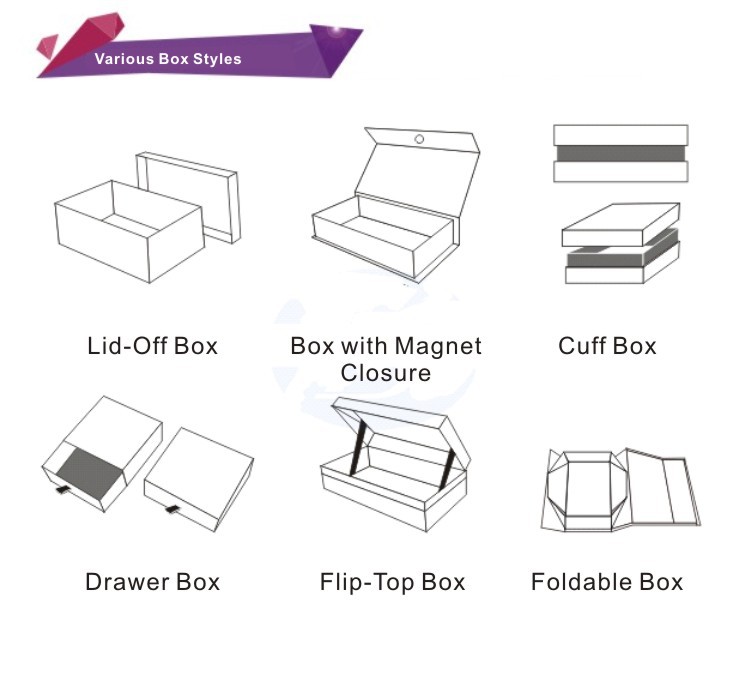The image showcases a detailed drawing of various box styles labeled in white text on a blue-purple background in the upper left corner that reads "Various Box Styles." The drawing features six distinct black-and-white illustrations of different boxes arranged in two rows of three. Each box type is represented by a clear, detailed drawing with its respective name written underneath in black text. In the first row, from left to right, are the "Lid Off Box," which is depicted with its lid removed; the "Box with Magnet Closure," showing a lid attached by a central magnet; and the "Cuff Box," featuring a detachable lid that snaps securely onto a partially cut box. The second row includes the "Drawer Box," represented by a box that slides open; the "Flip Top Box," which has a lid attached with a string mechanism to open and close; and lastly, the "Foldable Box," shown as a box that can collapse or fold. Each drawing accurately represents its function and design characteristics.